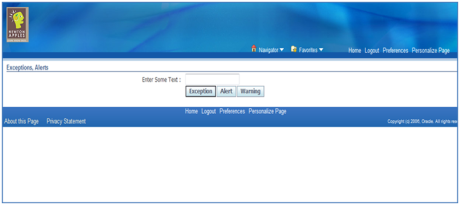This is a screenshot of an old web interface that appears to date back to the early 2000s, likely from the era when Netscape browsers were prominent. The image is landscape-oriented, featuring a rectangular box with a thin blue border and a prominent blue banner at the top adorned with some shading.

In the upper left corner of the banner is a brown rectangular logo that is somewhat blurry, making the text difficult to read. The logo appears to be part of a two-word company name and includes a yellow face oriented to the right. Around the face's ear area is additional coloring, and above the head are lines indicating the person is having an idea. 

The banner prominently displays the text "Exceptions Alerts." Below this is a horizontal line, beneath which the text "Enter Some Text" is displayed alongside a textbox for user input. Below this section are two buttons, labeled "Exceptions Alert" and "Warning." The term "Exceptions" is highlighted in bold.

At the bottom of the interface is another blue rectangle containing several hyperlinks: "About This Page," "Privacy Statement," "Home," "Logout," "Preferences," "Personalized Page," and a copyright notice that is too blurry to read entirely but appears to be from the early 2000s. 

Overall, this interface harkens back to the days of early web design, characterized by basic interactivity and straightforward layouts, suggesting it fails from a time when the internet was transitioning into a more user-interactive platform.